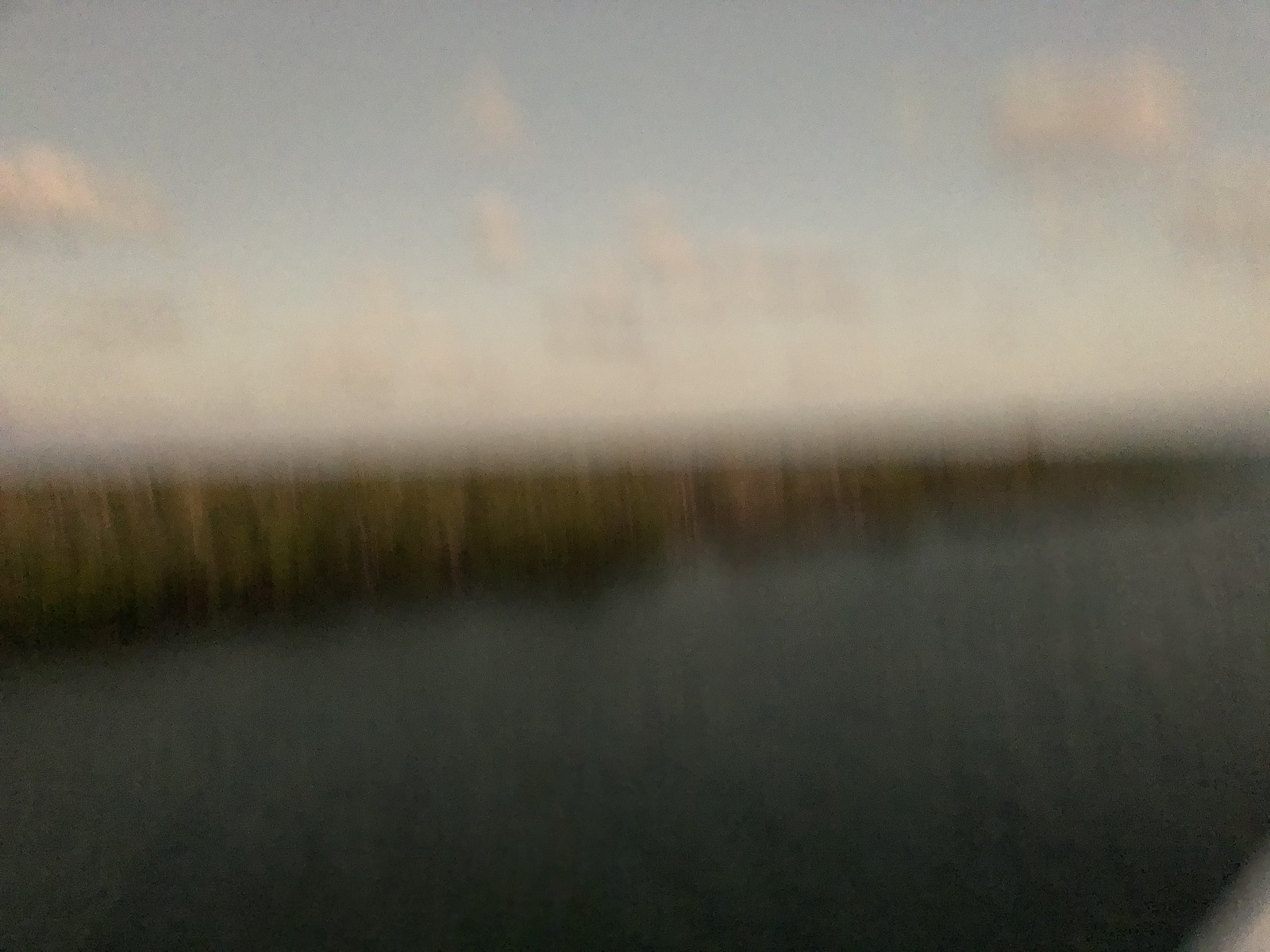The image is an extremely blurry, out-of-focus photograph that seems to capture a landscape divided into three distinct horizontal sections. The upper half of the image features a light blue sky scattered with fluffy white clouds, suggesting early sunrise. Below this is a narrow band that appears to be tall grasses, colored in shades of brown and yellow. The bottom section of the image is a deep bluish-gray, which could be interpreted as a body of water, such as a canal, creek, or river, or alternatively, a cleanly paved road. The blur gives the photo an oil painting quality, and it is likely taken from inside a moving car, as suggested by the even blur and the indistinguishable white object or roadside element seen in the bottom right-hand corner. The foreground vegetation appears swampy green and the entire scene gives an impression of a vast, open plain.